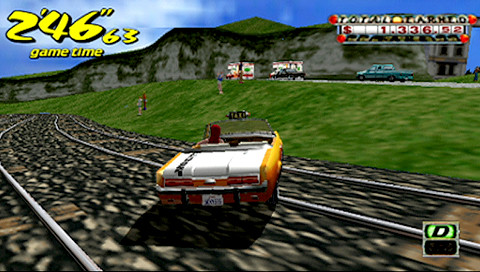This detailed, horizontal screenshot from the classic Sega Dreamcast game "Crazy Taxi" captures an intense driving moment. The scene is viewed from a third-person perspective, showcasing a yellow and white convertible taxi in the center of the image, seemingly veering off a rocky, rail-like track onto a small grassy hill. The track, resembling one made of large block rocks and pebbles, stretches from the lower right-hand corner to the middle of the left-hand side. The car’s driver, wearing a red hat, is navigating towards a green hill with a backdrop of distant grayish mountains and a vivid blue sky dotted with white clouds. Prominently displayed in the top left corner in yellow font with black shadows, the game time reads 2'46"63. The upper right corner shows the fare total of $1,336.52 in red numbers on a rectangular sign with red circles at the corners. Below this, a blue pickup truck is seen driving on another road towards the left side of the frame. The scene captures the exhilarating, chaotic essence of "Crazy Taxi" gameplay.